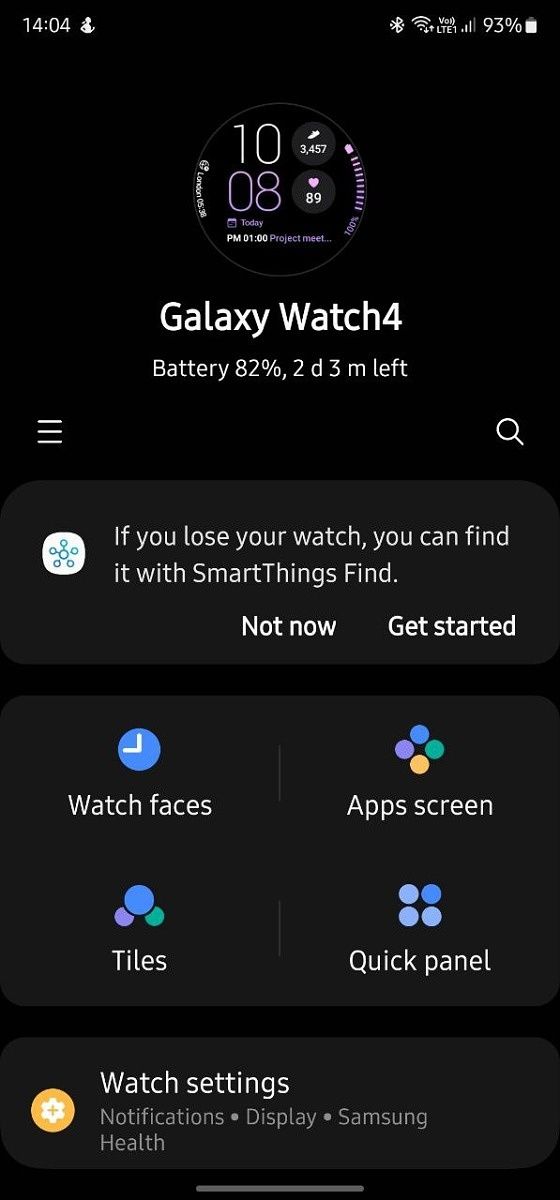This image is a screenshot taken on a smartphone. The time displayed in the top left corner is 14:04, while various status icons, along with a battery level indicator showing 93%, are visible on the right side of the screen. Below the time, the display shows the number "1008," which may be indicative of a date or another type of numerical identifier. Surrounding this are various other digits, contributing to the intricate display.

The center of the screen prominently features information about a Galaxy Watch. It includes the text "Galaxy Watch 4" along with the battery status noted as "Battery 82%", and an estimated usage time of "2d 3m left." Additionally, it states, "If you lose your watch, you can find it with SmartThings Find," providing options for "Not Now" and "Get Started."

Below this central section, there are four large icons, each contained in its own quadrant. The top-left icon, labeled "Watch Faces," features a clock image. The top-right icon is titled "App Screen" and shows four differently colored circles grouped together. The bottom-left icon, named "Tiles," displays a large circle with two smaller circles branching off of it. The bottom-right icon, titled "Quick Panel," consists of four circles arranged side by side.

At the bottom of the screen is an additional set of information and icons against an orange circular background that resembles a flower. It reads "Watch Settings," followed by icons and labels for "Notifications," "Display," "Samsung Health," and other relevant settings.